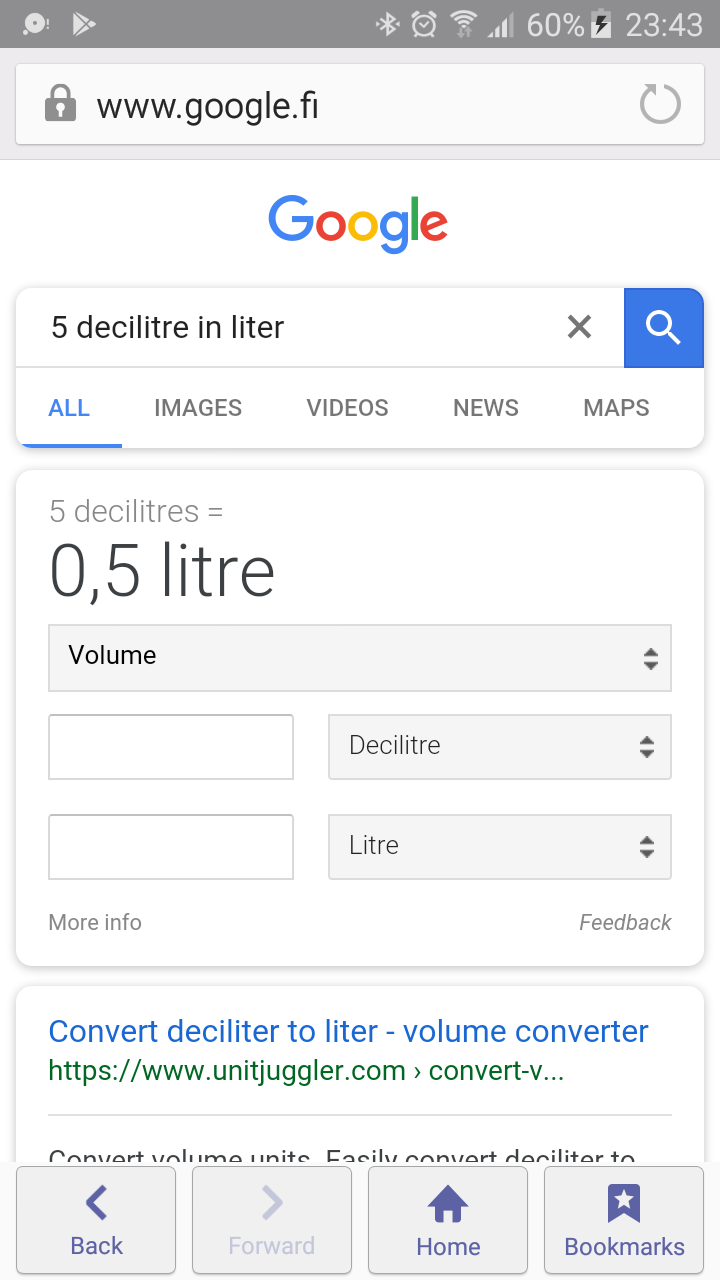This image is a detailed screenshot from a phone showing a Google search result for converting 5 deciliters to liters. At the very top of the screenshot, a gray bar displays various phone status icons: the time (23:43), a battery icon at 60% and charging, network signal strength, Wi-Fi, alarm clock, Bluetooth, and Google Play symbols. Directly below this bar is the URL bar indicating the search is being performed on the Finnish version of Google (www.google.fi), along with a lock icon on the left and a reload button on the right.

The main content of the screenshot is the Google search results page. The query entered is “5 deciliters in liters.” The page features several standard Google navigation tabs (All, Images, Videos, News, Maps), with "All" being highlighted. Dominating the center of the image is a Google calculator tool displaying the conversion result: "5 deciliters = 0.5 liters." This tool includes two blank fields for additional inputs. Below this calculator, a link leads to an external conversion website, unitjuggler.com, highlighted in green text, and labeled "Convert deciliter to liter volume converter" in blue.

At the bottom of the screenshot, the four main navigation buttons of the phone's browser are visible: Back (highlighted in blue), Forward (grayed out), Home (highlighted), and Bookmarks (highlighted). The overall color scheme of the interface is white on gray, ensuring clarity and ease of reading.